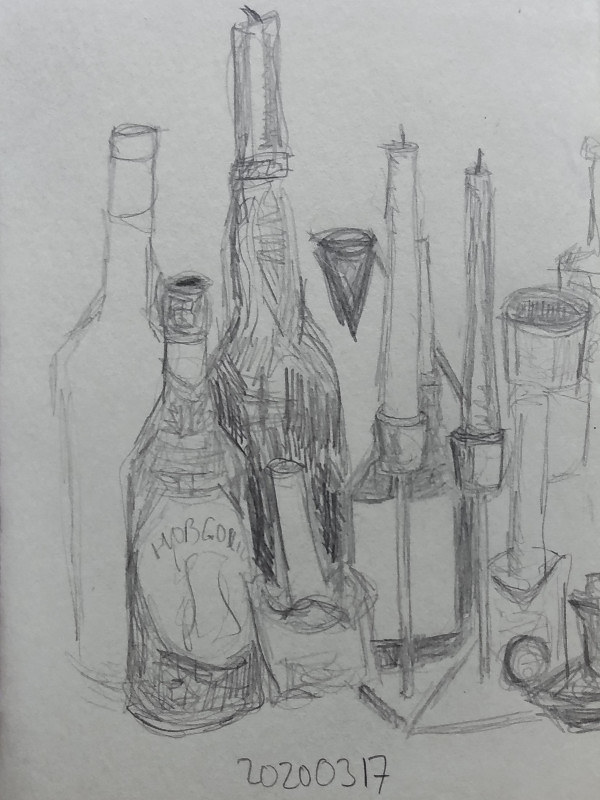This is a detailed pencil sketch depicting a group of bottles and candlestick holders. On the left side of the composition, three bottles of varying heights are arranged together. Two of these bottles are shaded in with meticulous pencil strokes, while the third remains outlined but unshaded, allowing it to sharply contrast with its counterparts. To the right of the bottles, there are four candlestick holders, each with a candle, standing proudly. The entire scene is drawn with a careful attention to texture and light. The artwork is dated "2020-03-17" at the bottom, marking its creation.